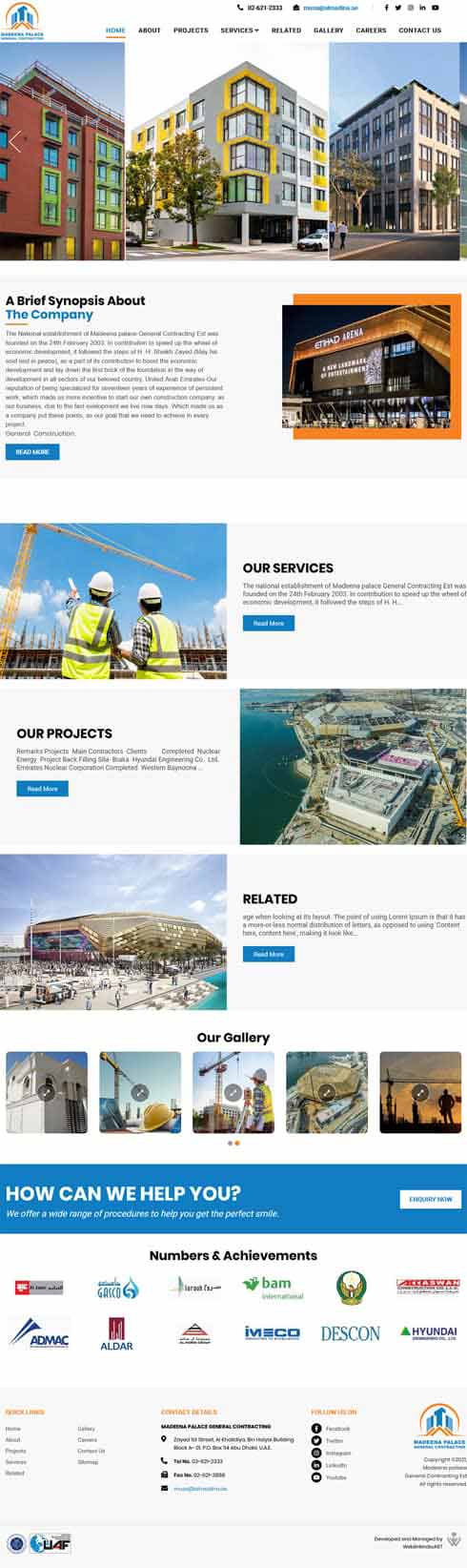This screenshot showcases a vertically elongated and visually cluttered website displayed on a desktop screen. The text and images appear very small and compact, making detailed content difficult to discern. Despite the reduced readability, the layout indicates a significant number of images—no fewer than 11 or 12—spread throughout the page.

At the top of the screenshot, various browsing buttons typical of a desktop interface are visible. The page prominently features different sections, beginning with a display of apartment listings accompanied by a brief company overview, although the text is too minuscule to read.

Below this introductory section, there is an image of two construction workers under the heading "Our Services," followed by some unreadable text. Further down, another image depicting an urban environment is labeled "Our Project." Adjacent to this section is an area titled "Related," showcasing a gallery of selectable images.

Toward the bottom of the website, a blue banner stands out with the text "How can we help you?" and a button presumably intended for users to send questions or inquiries. Finally, a series of logos representing the company's achievements are displayed, rounding out the webpage's content.

Overall, this website seems to be designed to showcase a company's services, projects, and achievements, though the extremely small text and images detract from its usability and visual appeal.